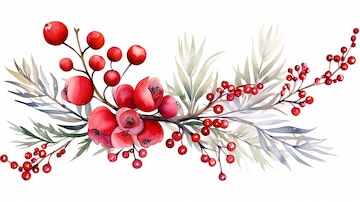This is a detailed drawing of a delicate mistletoe plant. The central branch, depicted in a browny-gray color, runs horizontally through the composition, serving as the anchor for the rest of the elements. Radiating from this branch are a series of relatively long, thin-shaped leaves. These leaves exhibit light, pastel shades of green and blue, with hints of dark green, contributing to the overall light and airy appearance of the mistletoe.

Scattered along the twig are small, round, berry-like fruits in vibrant shades of red and pink. These berries vary in size, with some medium to large ones appearing slightly opened, resembling rose buds, and suggesting they could potentially bloom into flowers. The smallest berries can be found at the edges of the mistletoe. 

Against a clean white background, the intricate details of the plant are clearly visible, emphasizing the contrast between the bright berries and the softer hues of the leaves. There is no text present in the image, allowing the viewer to fully appreciate the beauty and delicacy of the mistletoe illustration.